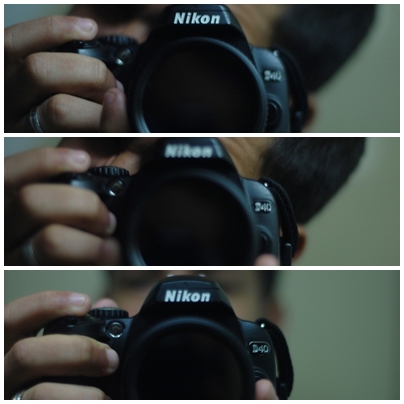This is a color photograph presented in a square format, composed of three stacked images in a column, all featuring a close-up view of an African-American individual with short black hair, holding a Nikon D40 camera. The top image shows the person with the camera up to their eye, preparing to take a photo, and you can see their fingers poised on the shutter button. The image focuses sharply on the camera's lens, which points directly at the viewer, while the individual's face is mostly obscured. The middle image captures a similar scene but with the Nikon logo slightly blurred and a model number partially visible, though illegible. The camera strap and the large lens are also noticeable. The bottom image shows the Nikon D40 logo clearly, with the same hand positioning as in the previous shots. The light gray background serves as a consistent backdrop throughout all three images.